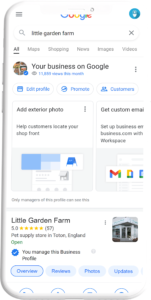The image features a detailed and dynamic interface set against a purple background. At the top of the image, there are three small black lines. The iconic Google logo, with its signature blue, red, yellow, and green colors, is prominently displayed, accompanied by a small mark above it. 

On the right side, a blue circle with a down arrow is visible. Just beneath it is a search bar containing the text "Little Garden Farm" with a magnifying glass icon on the left and an "X" on the right. Below the search bar, there are several tabs: "All" (which is underlined), "More," "Shopping," "News," "Images," and "Videos."

Further down, a circle contains a picture and a small blue circle with a check mark, along with the text "Your business on Google." Below this, some blueprint-like text can be seen, followed by three dots.

Next, there are three buttons: "Edit Profile," an unclear second button, and "Customers." A purple box labeled "Add Exterior Photo" with three dots is followed by text prompting customers to "help customers" with your shop front. 

The image also includes several smaller elements like pictures, three blue blocks, and a small blue top on an unspecified item. On the right, there's a prompt for "Get Custom Emails" along with a box containing the letter M and the letters D and O in the colors blue, red, yellow, and green. 

Underneath, another box displays "Little Garden Farm" with a blue circle and check mark, and a pictorial icon alongside three dots. At the bottom, there are buttons labeled "Overview" and another unclear option, as well as icons for phone and update. Additionally, there are four partially visible semicircles at the bottom of the image.